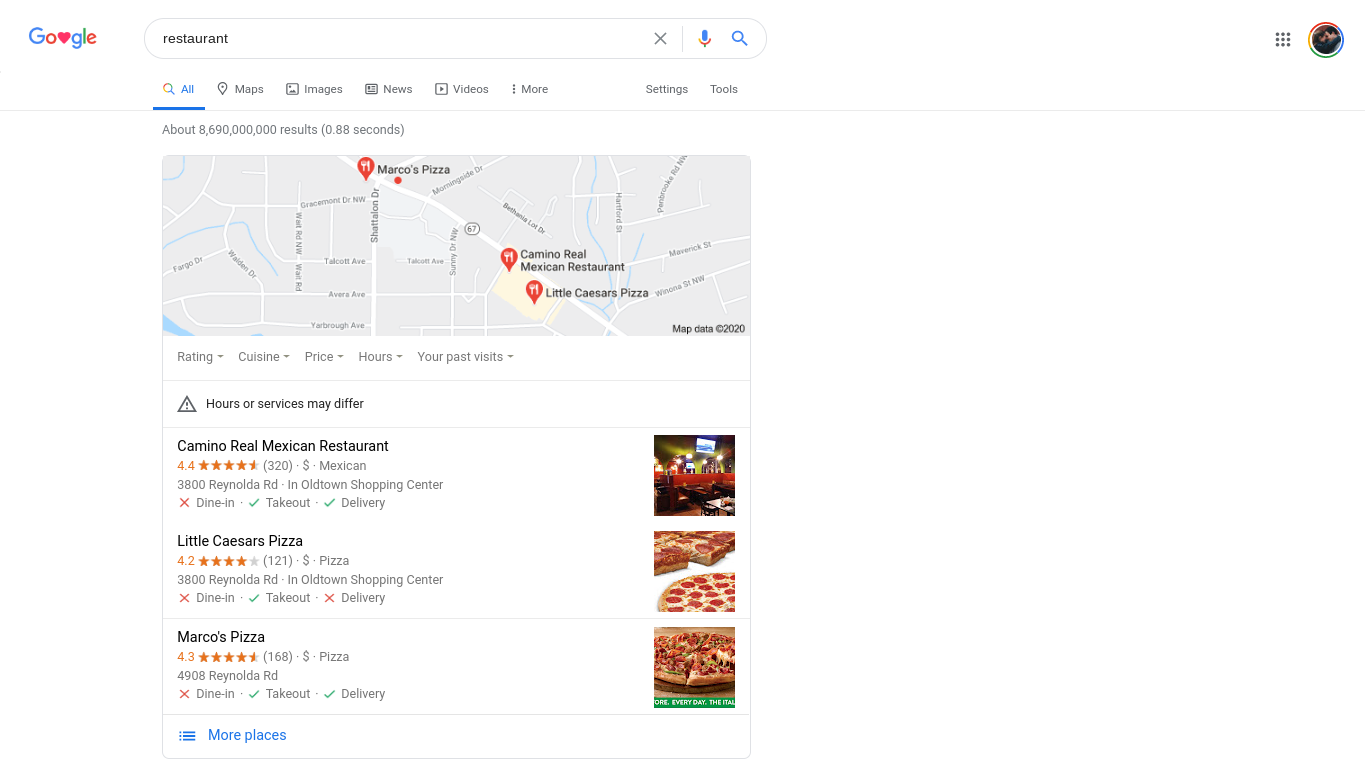The image depicts a Google search results page with "restaurant" as the query in the search bar. At the top left, the Google logo is visible, with the second 'O' stylized as a heart. To the right is the search bar containing the term "restaurant," alongside icons for clearing the search (X), voice search (microphone), and executing the search (magnifying glass).

Below the search bar, several tabs are present: "All" (currently selected and underlined), "Maps" (with a map icon), "Images" (with an image icon), "News" (with a news icon), "Videos" (with a video icon), and "More" (represented by three dots). There is also a settings tool icon.

The map section features a Google map with three pins indicating the following locations:
1. **Marco's Pizza** 
2. **Camino Real Mexican Restaurant**
3. **Little Caesars Pizza**

Additional details are provided for each restaurant:
- **Camino Real Mexican Restaurant**: Rated 4.4 stars based on 320 reviews, it offers Mexican cuisine at a moderate price ($). Located at 38 Reynolds Road in the Old Town Shopping Center, it supports both takeout and delivery options. There is an image of the restaurant interior.
  
- **Little Caesars Pizza**: Rated 4.2 stars with 121 reviews, known for its economical pricing ($). It is also located at 38 Reynolds Road in Old Town Shopping Center. Little Caesars offers takeout and delivery services and has an image of a pizza against a white background.

- **Marco's Pizza**: This restaurant has the highest rating among the three, with 4.8 stars from 168 reviews. It offers pizza at a moderate price ($) and is situated at 4908 Reynolds Road. It supports both takeout and delivery services and includes an image of pizza against a brown background.

At the bottom of the section, there is an option for "More places." 

The streets on the map are not clearly readable, but the map is visually present. The detailed ratings, cuisines, pricing, addresses, and service options are highlighted for user convenience.